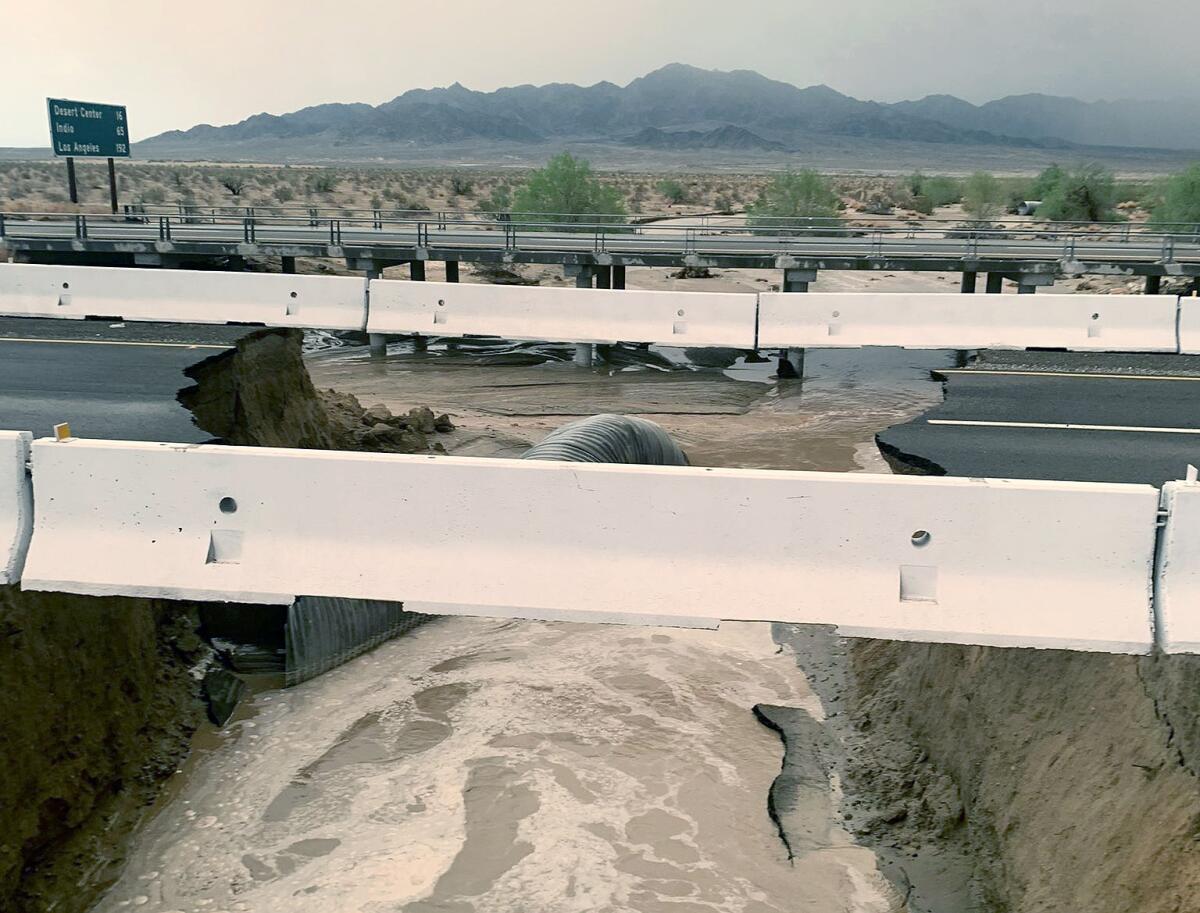The image depicts a dramatic scene of a partially destroyed bridge in a desert landscape. In the foreground, a decimated black roadway with white railings shows severe damage, with a significant section collapsed into a muddy, foamy expanse of water beneath. The water appears dirty, varying between gray and brown hues, and flows prominently down the center and left sides. The shattered road appears detached, with fragments submerged or seemingly vanished. Adjacent to this bridge, in the background, another bridge with thin bars is visible, also horizontally oriented but more intact. Amidst the desert backdrop dotted with green shrubs, a green directional sign reads “Desert Center 16, Indio 65, Los Angeles 152,” suggesting the scene is located in California’s Palm Desert area. Distant dark mountains under a partly foggy sky complete this strikingly clear and well-lit visual.